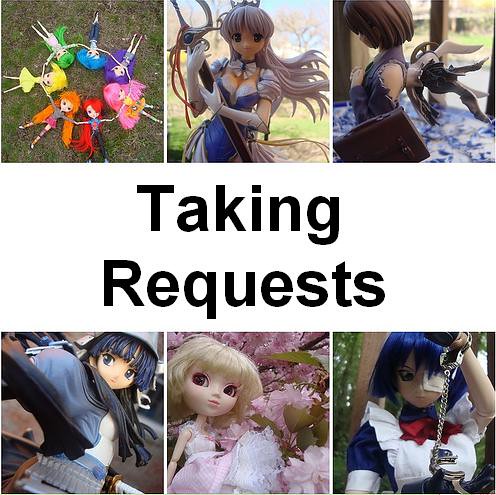The image comprises six small square pictures arranged in two rows of three, with prominent black lettering in the middle that reads, "Taking Requests." The squares feature animated doll-like figures. At the top left, there's a picture of several dolls dressed in varying colors of the rainbow, laying shoulder to shoulder in a circle. The top middle image showcases a doll with long blonde hair cascading down, seemingly holding onto a branch. To the right of that, there's a doll with short brown hair, appearing to have wings. The bottom row continues with three more doll images: the left one features a doll with long black hair, the middle one presents a doll with blonde hair dressed in pink, and the rightmost doll has blue hair and is depicted holding an object that resembles silver handcuffs or possibly a necklace. These intricate and colorful dolls create a visually appealing and whimsical collection.